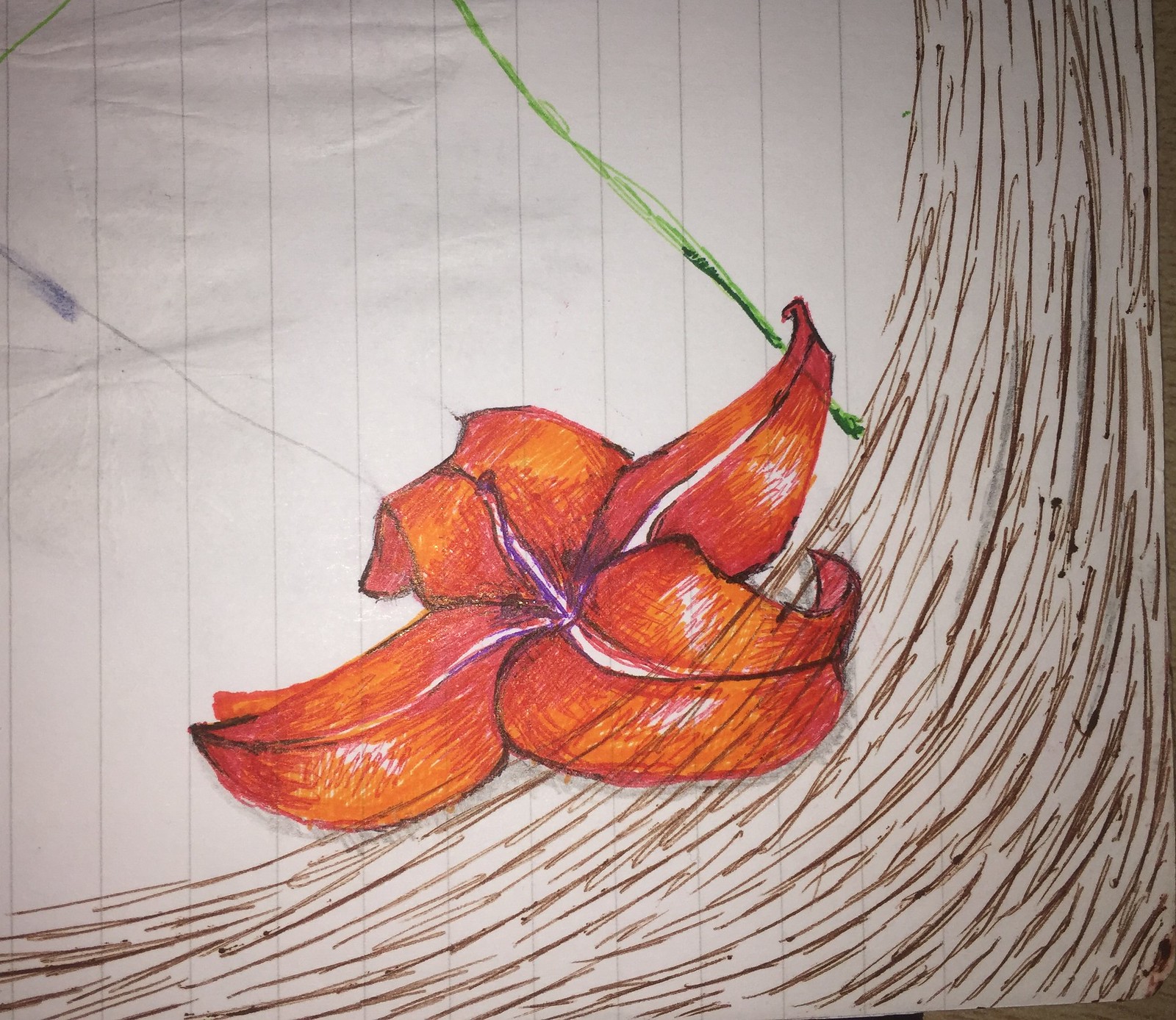This close-up photograph showcases an intricate piece of art rendered with colored pencils or ink. The focal point is an orange flower composed of four large, bisected, slightly curling petals. From the center of the flower, small, orchid-like purple formations emerge, adding an element of delicate complexity. The flower appears to be resting on a series of brown lines that streak and swoop from the upper right, curving downward to the left, reminiscent of cascading water, yet evoking the texture of tree trunks and roots stretching across the ground.

The artwork is drawn on lined paper, with minimal extraneous details distracting from the central elements. Notably, a green line extends from one side of the flower’s perimeter, not connected to it like a typical stem. Additionally, there's an errant gray line in the background, contributing to the piece's dynamic composition.